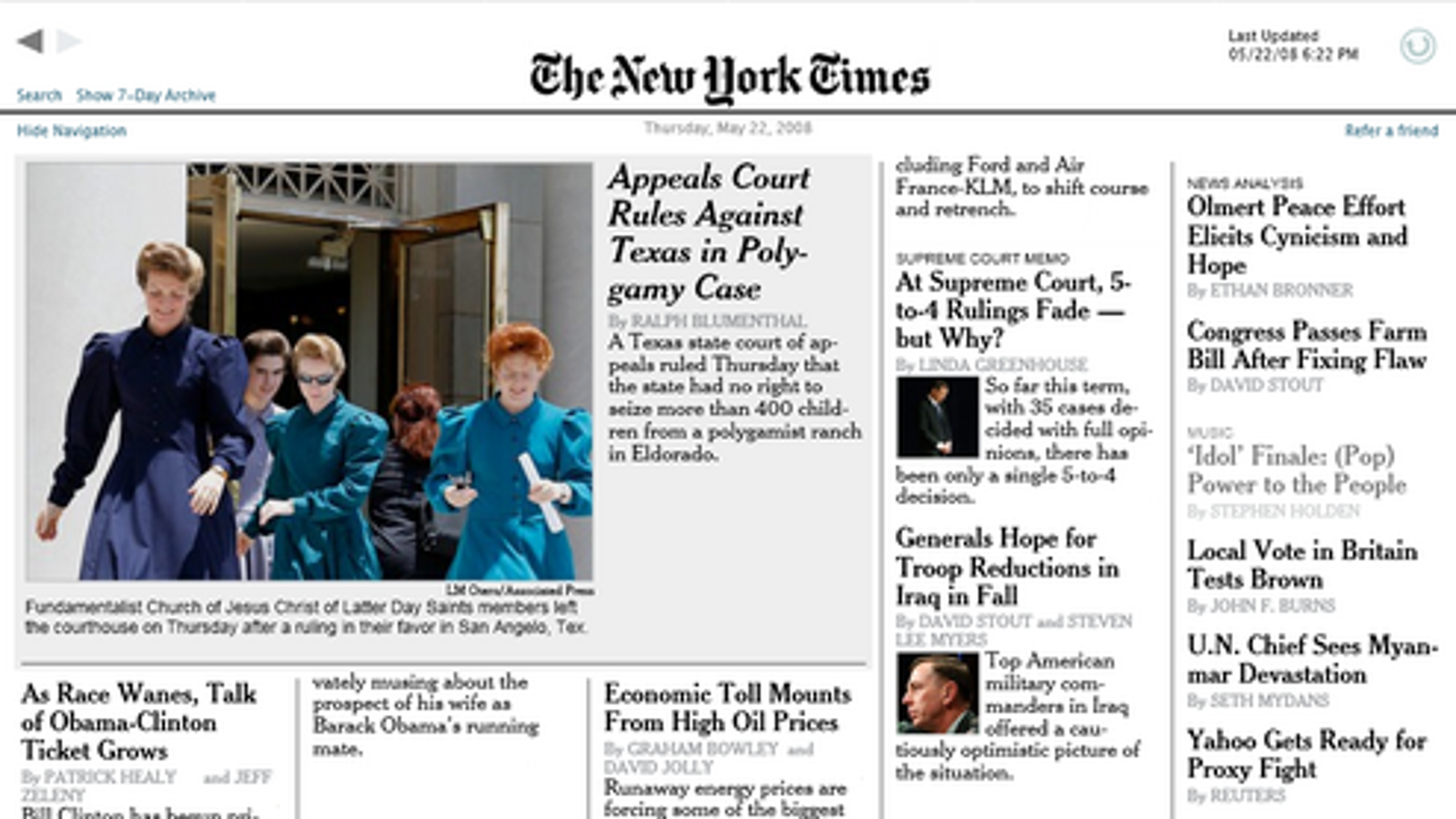This image, sourced from The New York Times, showcases a digital edition of the newspaper. The iconic "The New York Times" masthead is prominently displayed at the top center, featuring its traditional, ornate calligraphy-style font. Navigation buttons, including forward and back arrows, a search bar, a seven-day archive link, and an option to hide the navigation panel, are visible, indicating the digital nature of the display.

Beneath the masthead lies a headline accompanied by a poignant image. The headline reads, "Appeals court rules against Texas in polygamy case." The sub-headline explains, "A Texas state court of appeals ruled Thursday that the state had no right to seize more than 400 children from a polygamist ranch in El Dorado." The accompanying image captures members of the Fundamentalist Church of Jesus Christ of Latter-day Saints, dressed in bluish dresses with voluminous hairstyles, departing a courthouse following a favorable ruling in San Angelo, Texas.

Below this main story, additional articles are listed, complete with clickable links, offering readers an array of further reading options.